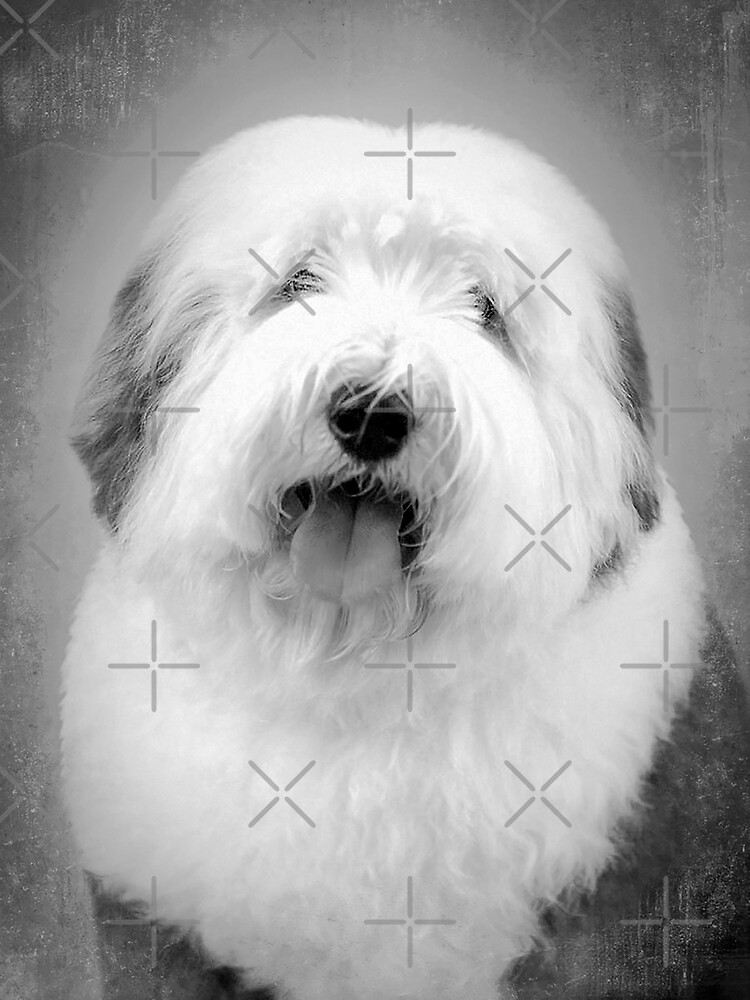This is a black-and-white close-up photo of a well-groomed sheepdog sitting on its haunches, centered in a vertical rectangular frame. The dog has a predominantly white, soft, and long-haired coat with darker grayish ears that have black tips, laid next to its head. Its face is mostly white, with long hair covering much of its eyes, which it peers through. The sheepdog's black button nose is framed by white shaggy hair hanging over the top. Its chest and shoulders feature a distinctive white bib that forms a V-shape, resembling a shawl, while the rest of its body shows darker gray fur. The dog's mouth is open, exposing its tongue, adding to the expressive, almost Santa Claus-like appearance. The background is blurred with shades of gray, and the entire image is overlaid with a pattern of gray X's and plus signs, giving it a creative, textured effect.